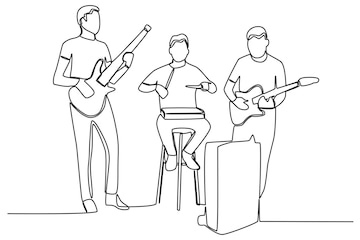In this simple yet detailed line drawing, rendered in very fine pen lines on a white background, three faceless men are depicted as band members on a stage. From left to right, the first figure stands holding a guitar, with short hair, a t-shirt, pants, and shoes visible. The middle figure sits on a stool, playing what appears to be a rectangular block or book, wielding two drumsticks. He is similarly clad in a t-shirt, pants, and shoes. The rightmost figure stands behind a small speaker or amp, absorbed in playing another guitar. Like his bandmates, he has short hair and wears a t-shirt and pants, but his legs and shoes are partially obscured by the rectangular box. The illustration focuses on the outlines of their bodies, clothing, and instruments, without any facial features.